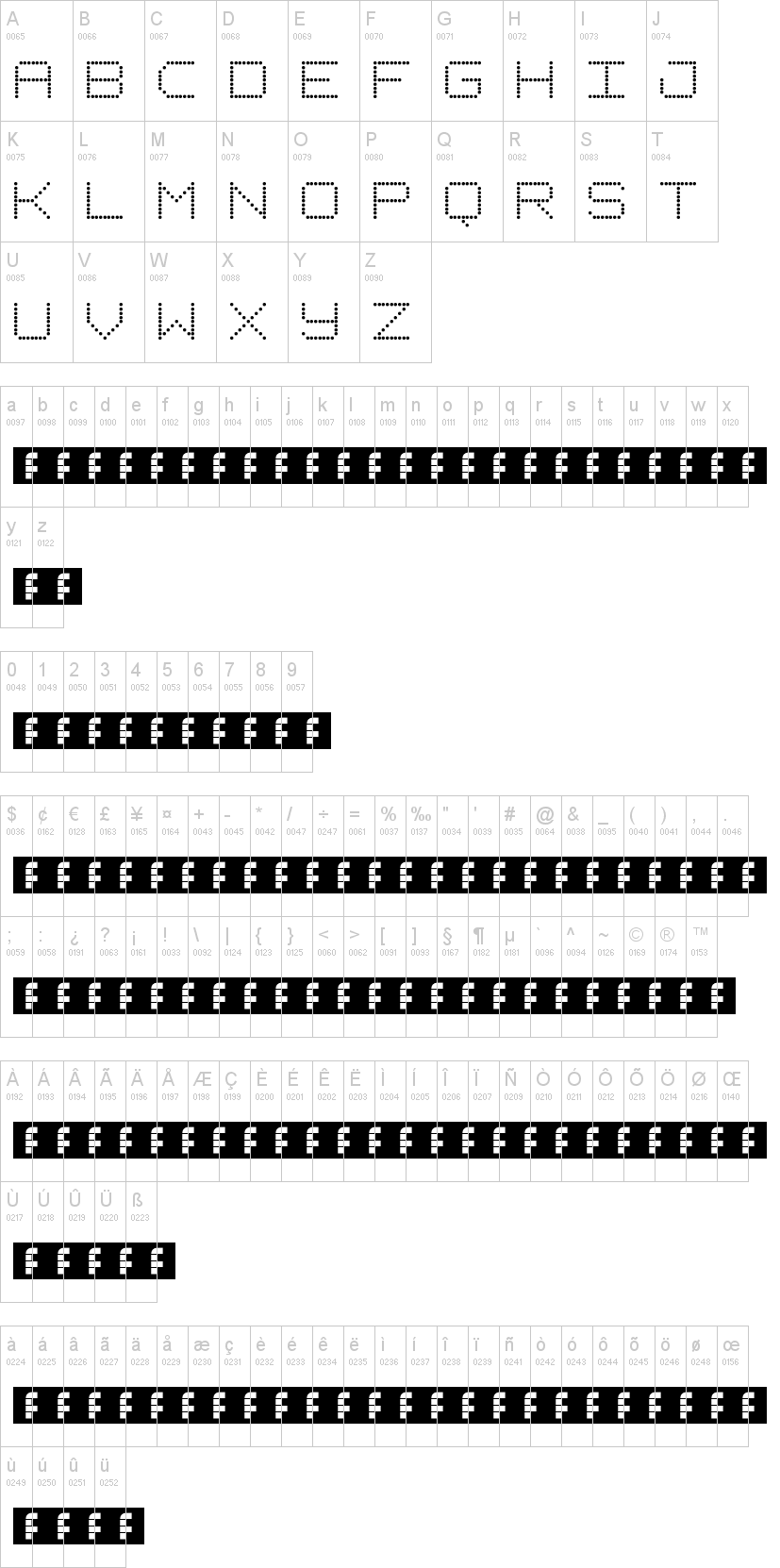The image is a detailed screenshot in portrait mode with a completely white background. Located in the upper left-hand corner are ten columns arranged in six rows. Each cell in these columns contains a letter represented in several formats: the letter itself, its hexadecimal value, and a dot matrix pattern.

In the upper left corner of the matrix, the letter "A" is displayed along with the code "0065" and a corresponding dot matrix. Adjacent columns follow the same format for letters "B" through "Z". For example, the cell for "Z" includes "Z," the code "0090," and its dot matrix representation.

Following these columns, there is a row starting again with "A," but this time, each letter has a different hexadecimal code, beginning with "A" as "0097." This sequence continues across the columns.

Below these rows, there is a notable long stripe with a black background. This stripe displays a repeated sequence of "FFF FFF FFF FFF FFF FFF FFF FFF FFF FFF," indicating a different kind of formatting pattern.

Further rows under this stripe follow the same repeated "FFF" pattern for various characters:
- Letters "Y" and "Z" follow with the code "FF."
- Numerical digits from "0" to "9" are displayed with all "FFF."
- Symbols from the dollar sign to a period, as well as characters from a semicolon to the trademark symbol, all have the "FFF" pattern.
- Uppercase accented characters from "À" to "Ç," letters "U" to a script-shaped "B," lowercase letters from "a" through "œ," and finally from "ü" to "ü" are all represented by the "FFF" pattern.

This image appears to display a comprehensive character set, including both standard and accented letters, symbols, and digit representations, all showcased in a combination of hexadecimal codes and dot matrix formats.